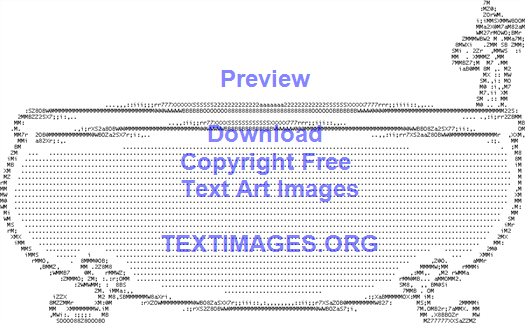This image, set against a white background, illustrates a bathtub created using ASCII art, a form of text-based digital art. The gray outline of the tub is composed of tiny, meticulously arranged dots forming dashed lines, which give it texture and shape. The bathtub has an old-fashioned design, characterized by curved rims and ornate legs at the lower left and right corners. On the upper right corner, the outline of a faucet, complete with handles, is visible. Overlaying this type-written art are several words in blue text: 'Preview' at the top, followed by 'Download', 'Copyright Free', and 'Text Art Images'. At the bottom of the image, 'TEXTIMAGES.ORG' is prominently displayed in all caps. These words are centered along the length of the tub and appear to be superimposed on the image, providing a clear call to action for accessing more such text art images.